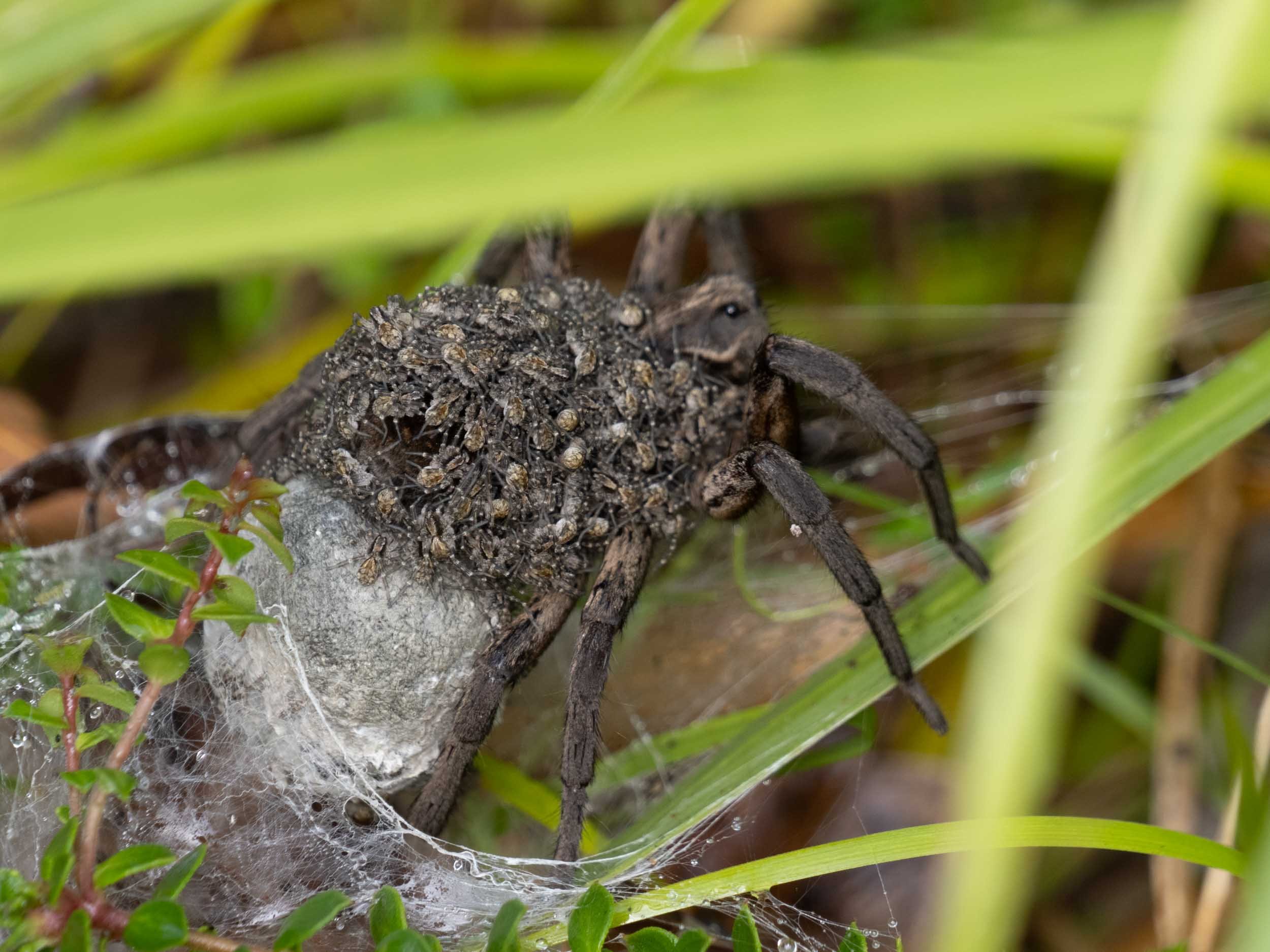In this detailed close-up image, a black and brown tarantula is the focal point, nestled amidst vibrant green grass blades and leaves that blur in the foreground and background. The tarantula, distinguishable by its distinct markings and sizable presence, is adorned with what appears to be hundreds of tiny spiderlings clinging to its abdomen. The mother spider rests on an intricately spun web, with a conspicuous ball of silk affixed to the lower part of her body. This visual marvel of arachnid reproduction accentuates the spider's maternal role while highlighting the natural web constructs around her. This image would undoubtedly evoke a strong reaction from anyone with arachnophobia, due to the sheer number of spiderlings and the spider’s imposing size.